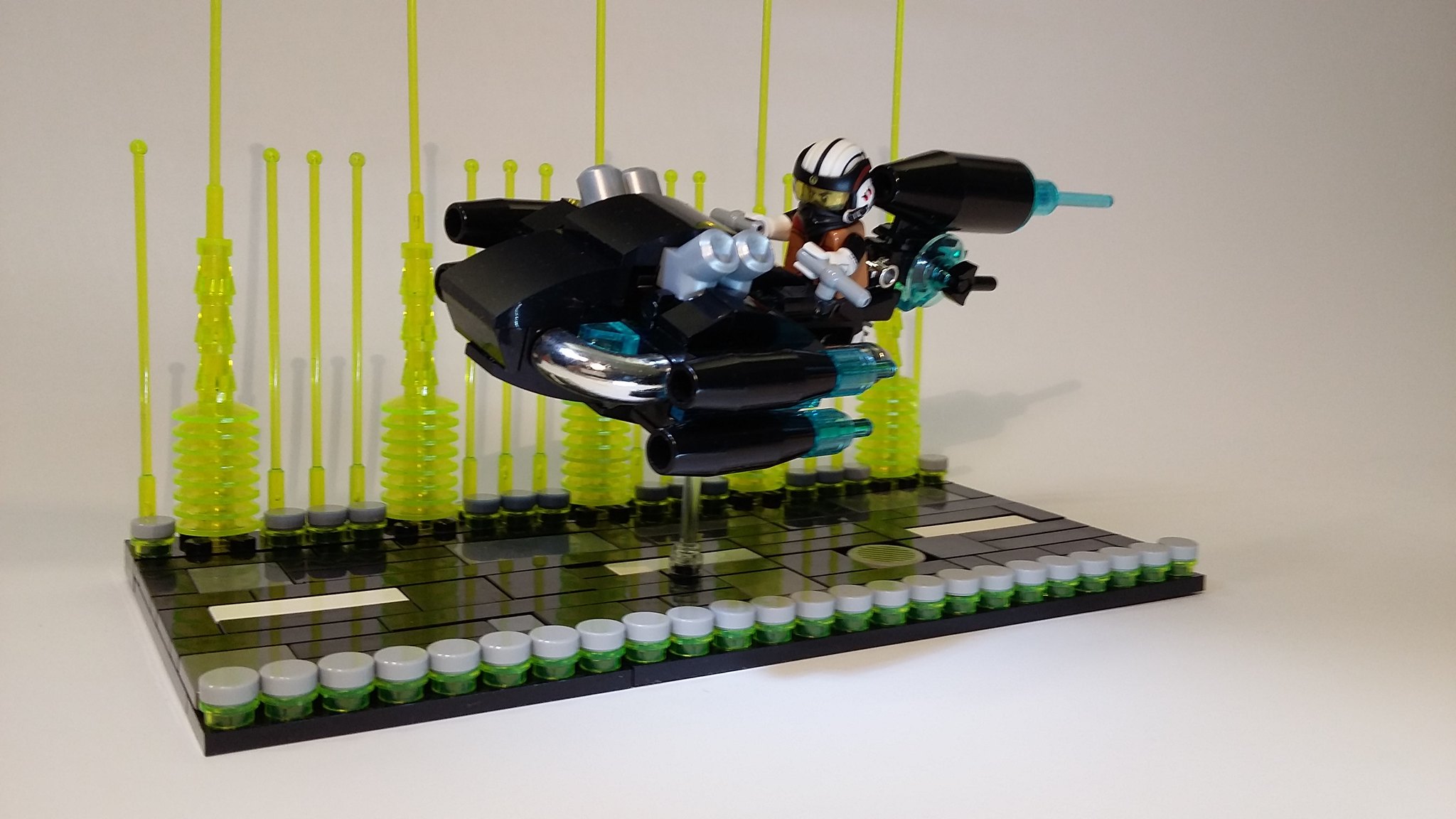The image depicts a detailed Lego sculpture of a black and silver spaceship, featuring a Lego figurine piloting it. The spaceship has distinctive silver thrusters and translucent teal pieces attached at the back, suggesting advanced propulsion. The cockpit is open, revealing the figurine wearing an orange suit with a black and white helmet, complete with a yellow visor. The pilot is seen grasping white throttle controls. Below the spaceship, which seems to hover, is a white tray lined with small jars containing a green substance, each sealed with a white lid. The background includes several neon yellow, translucent posts that reach the top of the image, which could be indicative of some sort of fueling or scientific apparatus. The entire scene suggests the spaceship is either flying over or displayed on a white surface with these additional features, possibly part of a larger Lego diorama or setup.